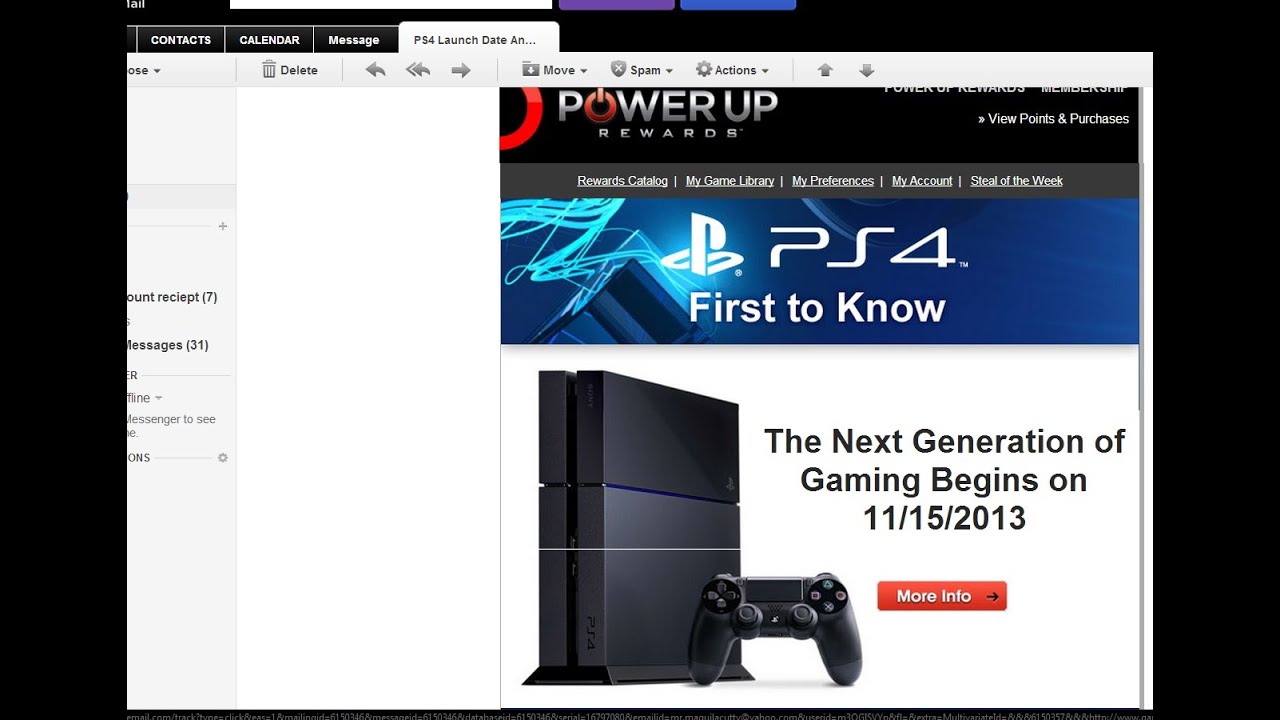This is a detailed screenshot of a webpage with a predominantly black background and a prominent white inset box in the center-right. The left margin of the page is partially cut off, revealing a gray sidebar with labels such as "Receipt (7)" and "Messages (31)", among other truncated entries.

At the top of the page, there are four visible tabs labeled "Contacts," "Calendar," "Message," and the highlighted tab "PS4 Launch Date." Below these tabs, several category options are displayed, including "Delete," "Move," "Spam," among others.

Central to the page is an advertisement for the PlayStation 4 (PS4). The ad has white text on a blue background, stating "First to know" beneath a technologically-styled blue squiggle and the iconic PlayStation symbol—comprised of a standing 'P' and an 'S' on its side.

At the very top of the inset box, there are sections titled "Power Up Rewards" featuring a large red half-circle on the left, and "Viewpoints" and "Purchases" on the right. Below these sections is an image of the PS4 gaming system. The console itself is gray, accompanied by a wireless handheld controller adorned with buttons and knobs for gameplay.

The advertisement proclaims, "The next generation of gaming begins on 11-15-2013," inviting users to click for more information.